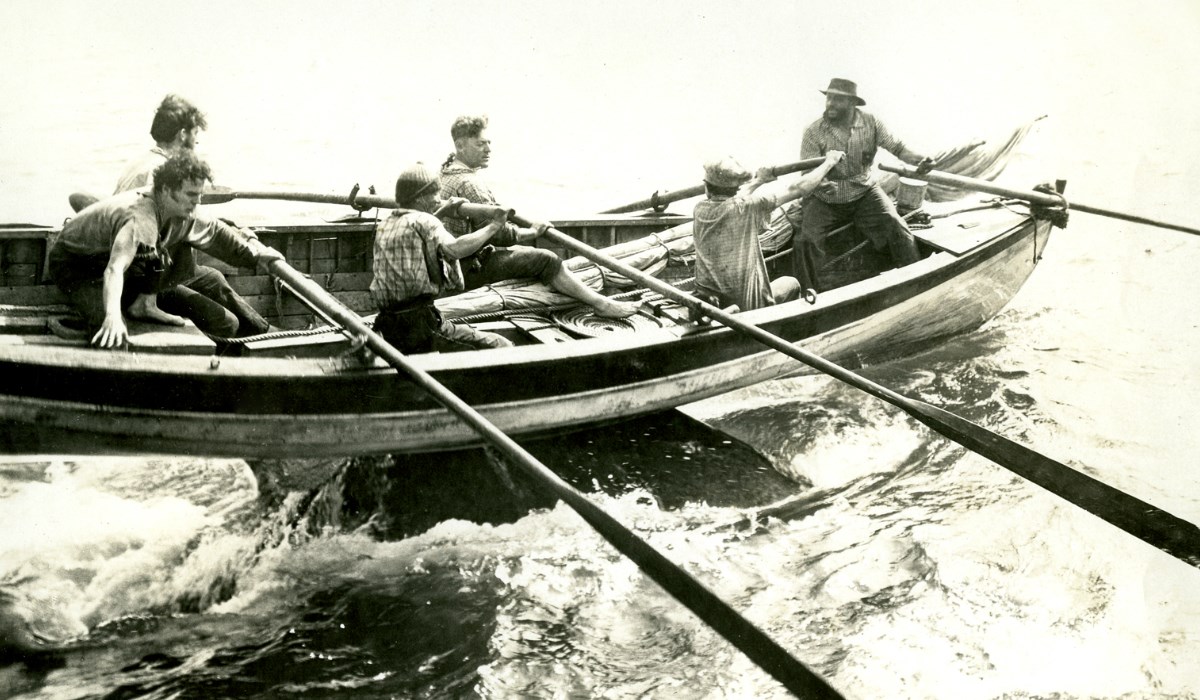This black-and-white photograph, slightly tinted yellow and overexposed, captures a dramatic moment of six individuals on a boat navigating rough waters. The boat is being lifted, possibly by an unseen force beneath, resembling a whale surfacing. All six individuals, dressed in collared shirts with jeans rolled up to their knees, clutch long oars, working together to row. Positioned across three rows, there are two men at the back, another middle-aged man and a teenage boy in the center, and at the front, a man wearing a top hat facing inward with a young boy around nine or ten years old by his side. The man in the hat appears to be shouting orders, adding to the scene’s intensity, as the choppy waves crest at the surface, highlighting their peril.